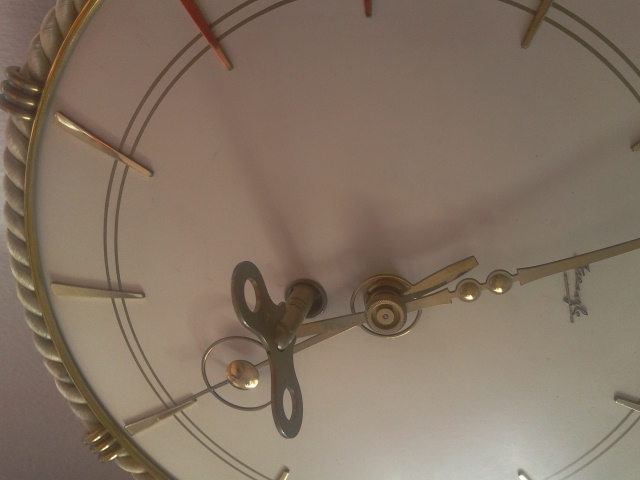This close-up image captures the face of a unique clock, seemingly taken from a side angle, causing the clock to appear as if it is lying on its right side. Notably absent are the traditional numbers, replaced instead by simple yet elegant lines marking each hour. The clock's outer edge features an intricate rope design, adding a touch of sophistication against the stark white face of the clock. Positioned just above the clock's hands is a small metal key, hinting at a winding mechanism and adding an element of intrigue to this otherwise minimalist timepiece.